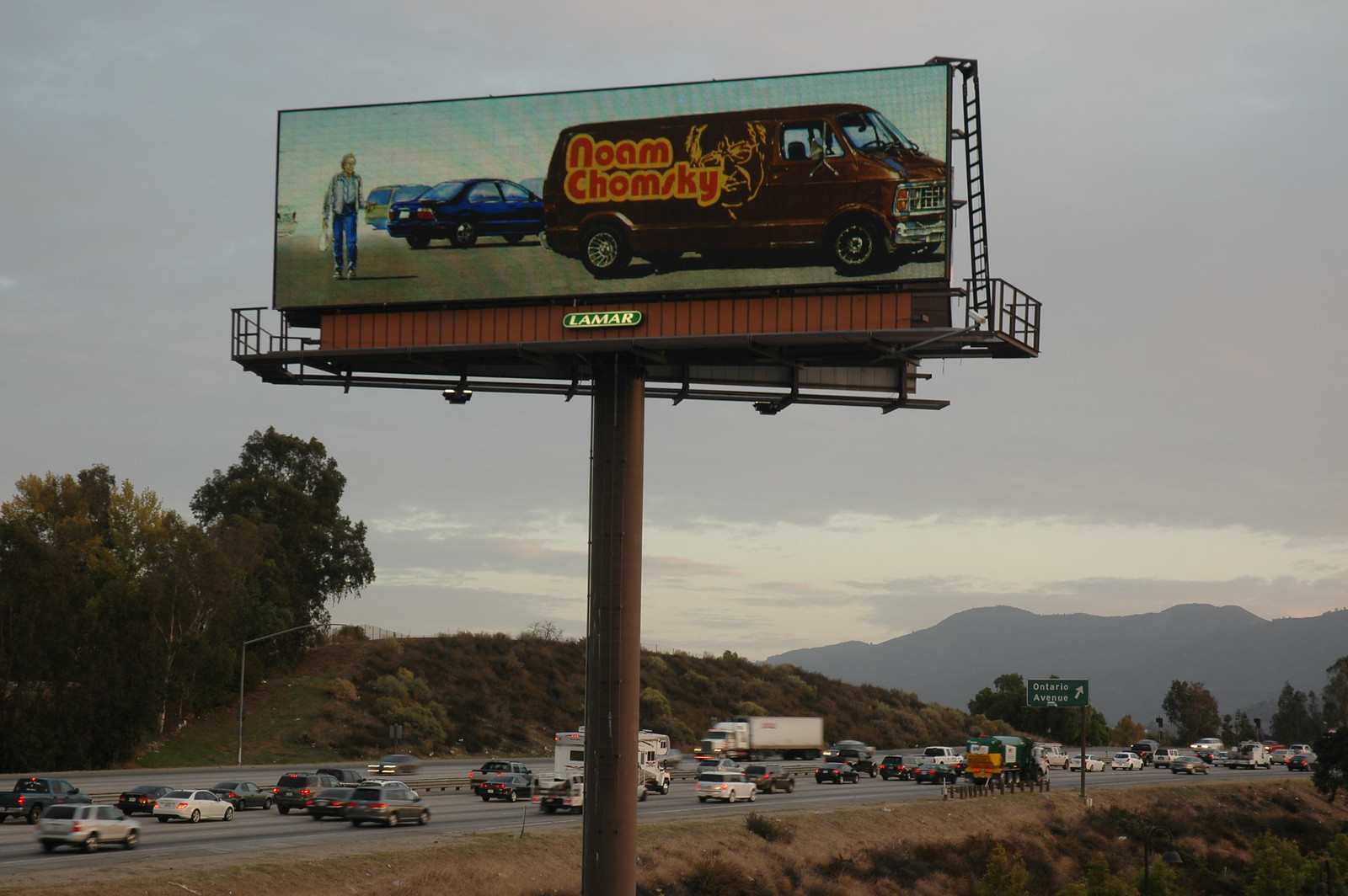This daytime photograph captures a detailed scene along a busy six-lane highway, bordered by fields, trees, and distant mountains beneath a cloudy, slightly bluish-purple sky. The highway, dense with various vehicles including passenger cars, SUVs, campers, and tractor-trailers, stretches from left to right with traffic flowing steadily.

In the foreground, a tall cylindrical brown support pillar lifts a prominent rectangular billboard. The billboard features a vintage 70s-style brown van parked in a busy parking lot, captured in profile. The van's side is emblazoned with "Noam Chomsky" in red lettering outlined in gold. Beside the van, a man is walking with a bag in his right hand and his left elbow bent. Behind the van, a blue four-door sedan is also visible.

The billboard's support structure is detailed with a green oval bearing white lettering that reads "Lamar," and a surrounding walkway featuring a ladder on the right side. Additionally, a directional road sign is visible near the highway, indicating "Ontario Avenue" with a white arrow pointing up and to the right. The scene combines elements of both urban infrastructure and rural tranquility, providing a rich, layered visual narrative.